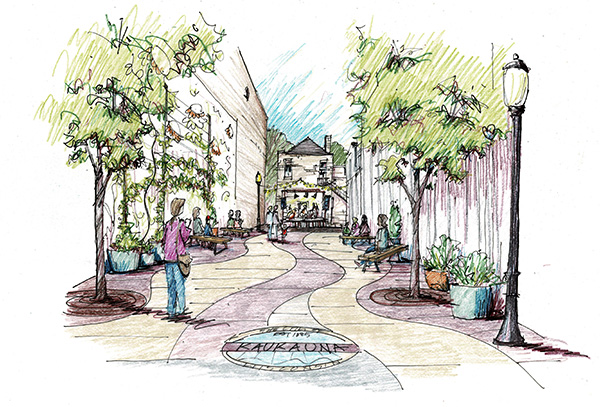This picture depicts a detailed, color pencil illustration of a lively downtown walking street. The street, marked by a blend of white and purple colors, features a central oval plaque with the text "KAU KAU NA." Trees with green leaves line both sides of the street, providing shade for people walking or sitting on park benches. On the right side, a prominent street lamp stands in the foreground, with another visible further down on the left. The background reveals a house at the end of the street under a partially blue and white sky. The busy scene includes various people, some seated on benches, and a woman standing under the shade, all contributing to the vibrant daytime ambiance. The sketchy style and abundant use of color pencils give the illustration a rich and textured appearance, capturing the essence of a bustling urban area.